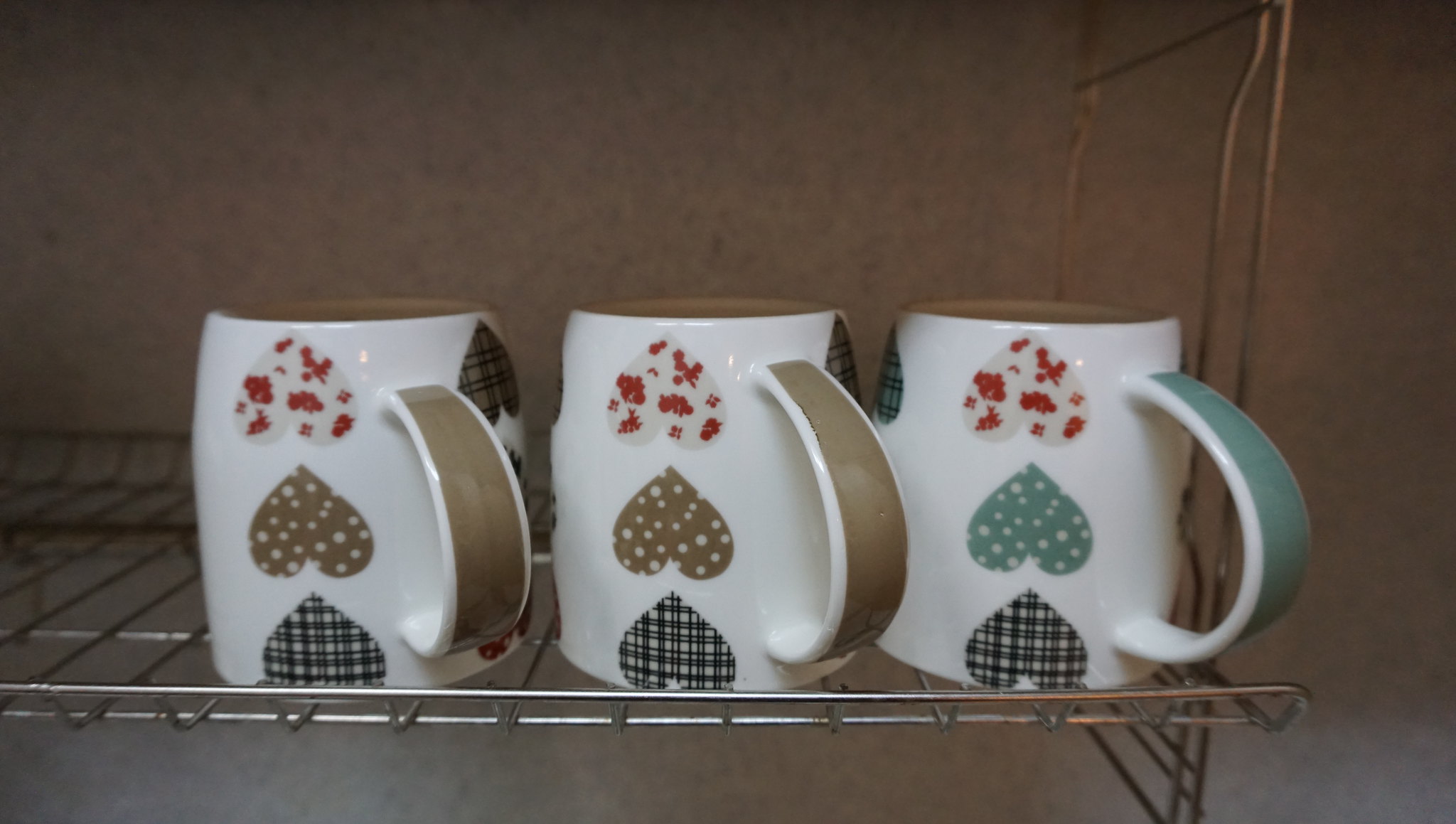The image depicts three ceramic mugs positioned upside down with their handles facing to the right, resting on a metal wire rack that is mounted on the wall. The wire rack, resembling a low-lying shelf with higher support wires extending upwards, might be placed on a brownish-gray countertop or a similar surface. The background features a nondescript, mottled wallpaper. Each mug is primarily white and adorned with three vertically aligned heart designs repeated around its surface. The hearts come in distinct patterns: one is red with a white background, another is brown with white polka dots, and the third is black and white plaid. Correspondingly, the handles of the mugs are colored to match one of the hearts—two handles have a metallic brown hue, and the third has a greenish-teal tint. This setup appears to be from either a personal kitchen or a restaurant, with no other objects or text present in the photograph.